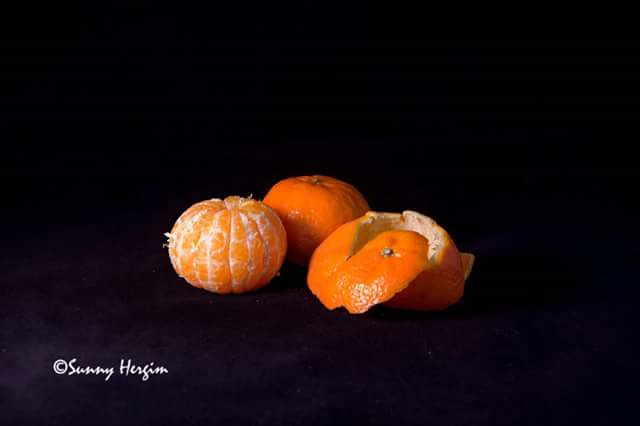This professionally taken photograph features a trio of clementines elegantly arranged on a solid black background, which may appear somewhat blurry due to potential quality loss during scanning. In the center, a fully peeled clementine reveals its glistening, pith-covered segments, while an adjacent unpeeled clementine sits at a slight angle to the right of the peeled fruit. A serpentine strip of orange peel, seemingly removed in a single, continuous piece, lies in the foreground, partially obscured by shadows. The soft light, entering from the left, delicately highlights the textures of the fruit and the peel. The scene is framed by a black, likely velvet, backdrop that enhances the focus on the clementines. In the bottom left corner, the copyright notice by photographer Sammy Hangen is inscribed in small, elegant cursive, adding a touch of personal craftsmanship to the carefully composed image.